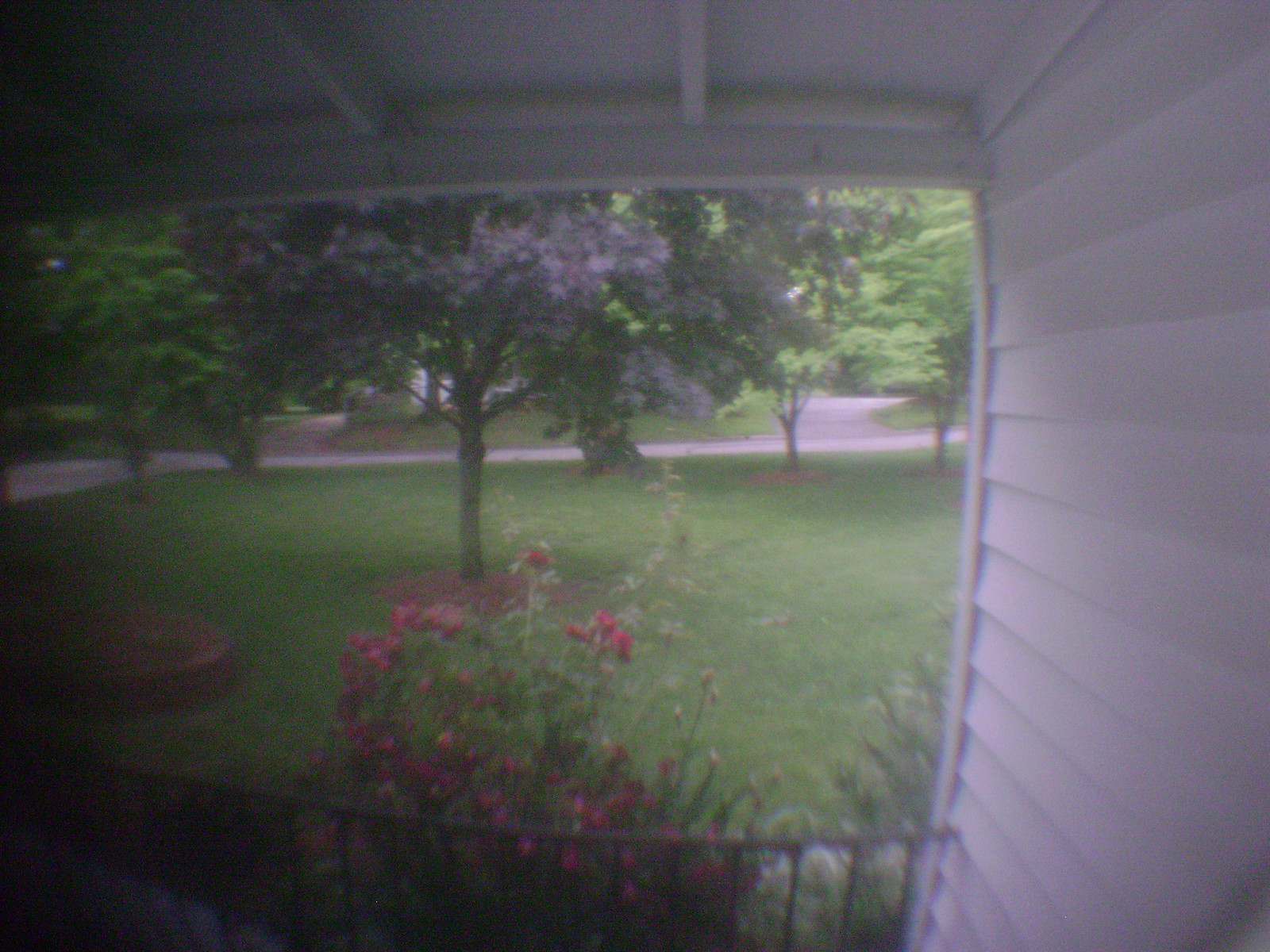Here is a cleaned-up and more descriptive caption based on the given input:

---

Captured by a security camera installed on the porch, this image reveals a serene outdoor space characterized by meticulously maintained features. The porch itself is framed by white siding and supported by white-painted rafters, creating a clean and inviting structure. A black railing, about three feet in height, runs along the porch's edge, offering a subtle yet functional barrier. Beyond the railing, a vibrant array of flower bushes showcases a delightful mix of red, pink, and yellow blooms, interspersed with lush green leaves. The foreground scene is completed by a well-manicured lawn of verdant green grass, which stretches out towards several young trees. Among these, a tree with striking purple leaves stands out, complemented by other recently planted trees with fresh, green foliage, contributing to the overall tranquility of the yard.